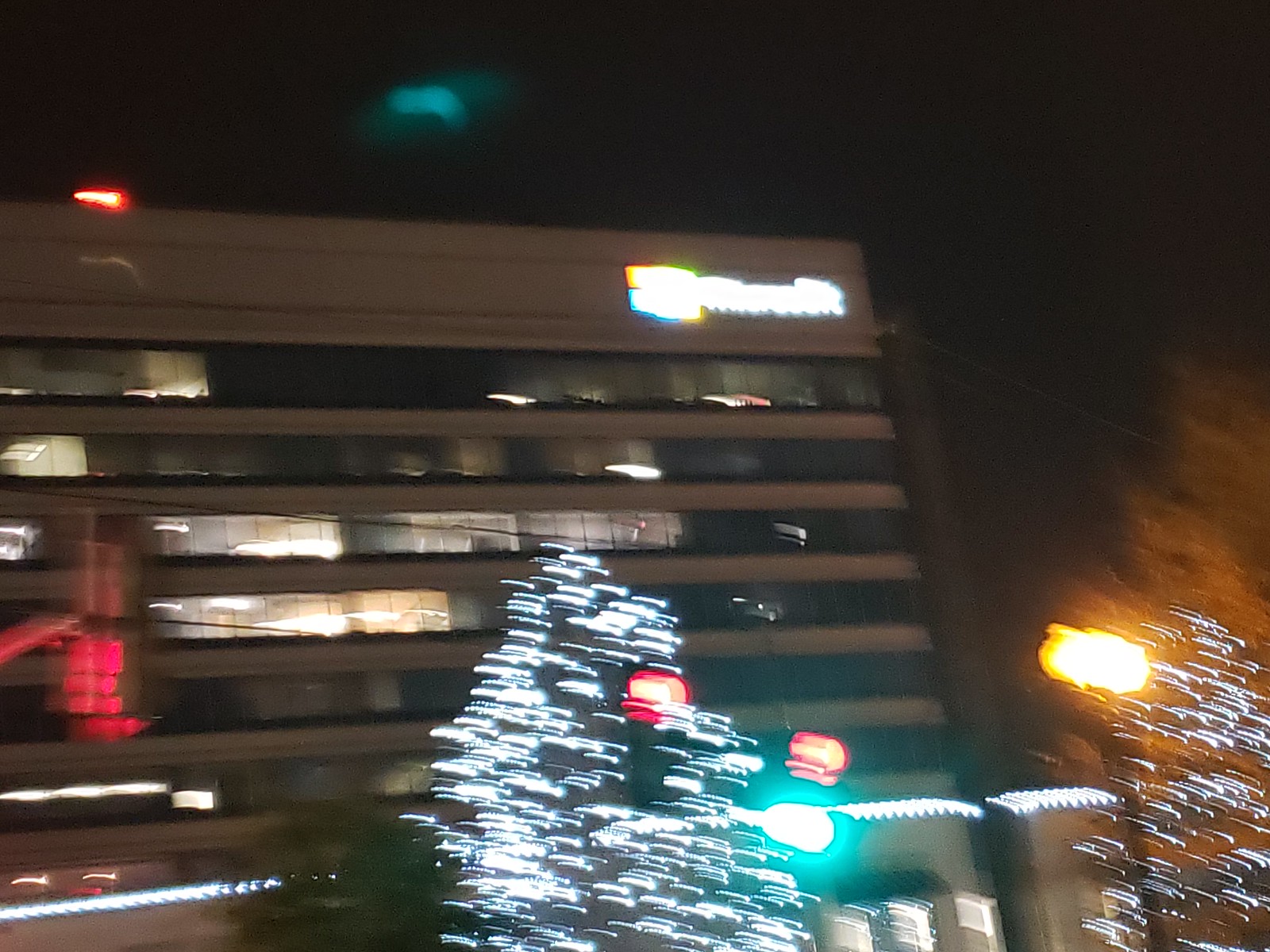This nighttime photograph captures a large gray building, identified as a Microsoft office due to the illuminated but blurry Microsoft sign and logo at the top. The sky is black, and the building's multiple floors are separated by gray horizontal lines. Many windows are visible, with about half lit by interior lights. At street level, several Christmas trees are decorated with lights. On the left, a tree is adorned with white lights, while on the right, a brown tree is partially lit with white lights. There are various streetlights and lamps, including a yellow light near the decorated Christmas tree, a green light beside the white-lit tree, and discernible red and green stoplights. Additionally, a white line of lights runs along the bottom edge of the building, adding to the festive ambiance.